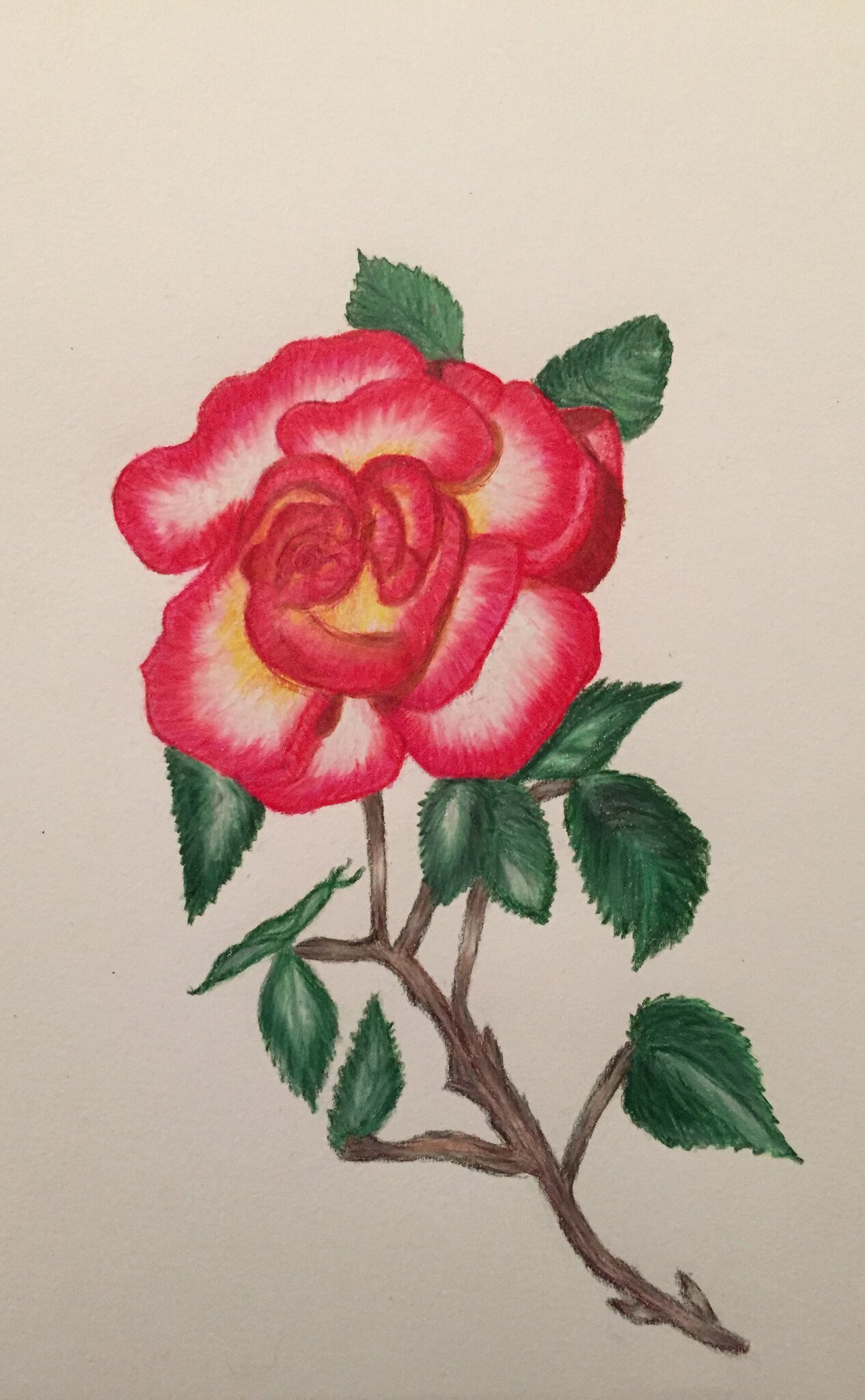This detailed sketch showcases a intricately drawn flower, starting from the bottom right-hand corner. The base of the flower is formed by a dark brown vine that extends diagonally to the left. Several smaller brown vines branch off from the main stem, each adorned with dark green leaves. A singular, prominent brown vine ascends and transforms into a beautifully shaded rose. The rose features pink petals accented with yellow spots towards the top and center. The innermost petals exhibit delicate white shading at their cores. Additional green leaves are present at the apex of the rose. The entire background is subtly colored in light gray, allowing the flower to stand out in striking detail.